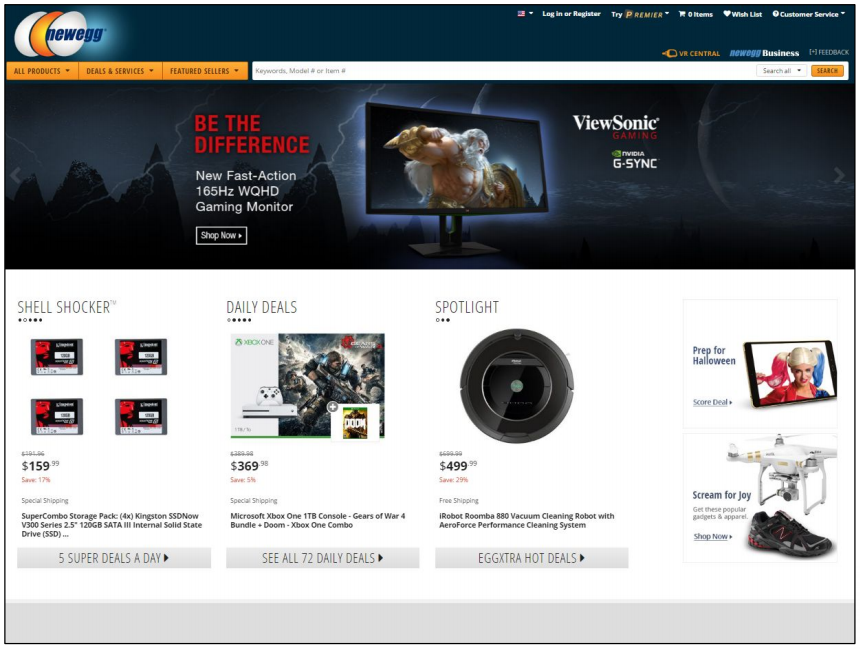This detailed caption describes a screenshot of a webpage, resembling the design and colors associated with Amazon.

The upper third of the image features a dark blue background. In the top left corner, there is the Newegg logo in lowercase blue letters, against a backdrop of three eggs—white, gold, and white. The third egg has a light blue glow around it and the word "newegg" over it.

To the right of the Newegg logo, there is an American flag icon for region or language selection. Adjacent to it are white text links for logging in or registering, followed by an orange link reading "try premier." Next to these links, there is a basket icon indicating "0 items," a heart icon labeled "wishlist," and a white circle labeled "customer service."

Below the Newegg logo, there are three orange tabs with black text: "All Products," "Deals and Services," and "Featured Sellers." Underneath these tabs is a white search bar with placeholder text in gray: "Keyword, Model, Number, or Item Number." On the far right of this search bar, there are two white buttons labeled "Search All" and "Search."

Beneath this section, there is an image showcasing black mountains and lightning bolts with the phrase "Be the Difference" in red text. Below that, in white text, it mentions a new fast-action 165Hz WQHD gaming monitor with a "Shop Now" call to action. The monitor displays game footage of a Zeus-like character, depicted as a muscular man with long white hair and beard, holding a shield with his left arm and clenching his fist with his right. To the right of this, the words "ViewSonic" in white and "Gaming" in red are displayed, along with "G-SYNC" in all-capital white letters.

The next portion of the image has a predominantly white background with a gray bar at the bottom. This section contains four columns:

1. **Shell Shocker**: Displays four game cartridges or packs with a red face, priced at $159.99 with a 1.7% discount. A caption reads "Special Shipping," "Super Combo Storage Pack," and details about a Kingston SSD V300 series 120GB internal solid-state drive with "Five Super Deals a Day."
   
2. **Daily Deals**: Features an Xbox One with a character in a black suit with blue lines. The package is priced at $369.98 with a 3% or 5% discount, including special shipping. The bundle comprises the Microsoft Xbox One, a 1TB console, Gears of War 4, and Doom Xbox One Combo. There’s a notice to "See also the two daily deals."
   
3. **Spotlight**: Displays a black Roomba priced at $499.99 with a 29% discount and offers special free shipping. The full title reads "iRobot Roomba 880 Vacuum Cleaning Robot with Air Force performance cleaning system." An "Eggstra Hot Deals" pun is visible here, using the "EGG XTRA" wordplay.
   
4. **Prep for Halloween**: Highlights a tablet featuring a person dressed as Harley Quinn with blonde hair styled in pink and blue ponytails. Below, there's an image of a drone accompanied by text encouraging viewers to "Scream for joy" and explore popular gadgets and apparel, urging them to "Shop Now." The drone hovers over what seems to be a black New Balance sneaker.